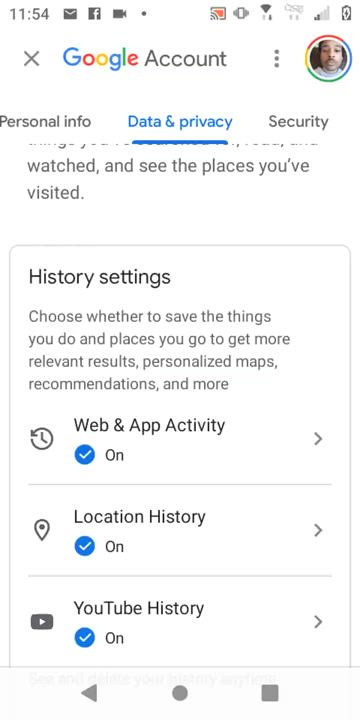The image displays a partial view of a web page, presumably accessed on a smartphone. At the top of the screen, the number "1154" is prominently displayed, followed by icons for email, Facebook, and video. The status bar indicates that the device is connected to the internet and the battery is either charging or has sufficient power.

Below this, the page title reads "Google Account," accompanied by a user profile image depicting a younger individual who appears to be either Hispanic or light-skinned African American. The page is divided into sections, with "Personal Info" highlighted at the top. Subsequent sections include "Data & Privacy" and "Security," providing an organized layout for managing account settings.

Further down, under "History Settings," there's a brief description instructing the user to choose whether to save their activities and locations to receive more relevant search results, personalized maps, and recommendations. The status indicators show that Web & App Activity, Location History, and YouTube History are all turned on. There are clickable arrows next to each setting, allowing the user to navigate deeper into these options.

Overall, the image encapsulates the user interface of a Google Account settings page on a mobile device, detailing various privacy and history settings the user can manage.